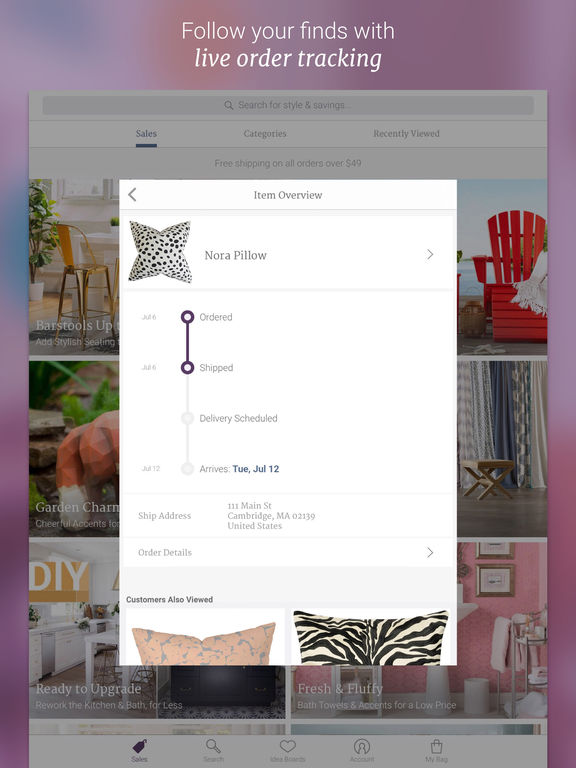In this screenshot of a shopping page specializing in furniture and accessories, the background fades into pastel hues of purple and blue, creating a soft and inviting atmosphere. Dominating the center is a white vertical rectangle that highlights the primary content of the page. At the very top, a header reads, "Follow your finds with live order tracking."

Within the white rectangle, labeled "Item Overview," is an image of the "Nora Pillow," a black-and-white polka dot cushion resembling a four-pointed star. The status of the order is prominently displayed: both "Ordered" and "Shipped" steps are darkened circles, linked by a continuous line, indicating that the item has been ordered and shipped. However, the delivery has not been finalized; this is depicted by a light gray line leading to a dimmed circle labeled "Delivery Scheduled" and another extending to "Arrives Tuesday, July 12th."

The text specifies that the Nora Pillow was shipped on July 6th, with further details including the shipping address: 111 Main Street, Cambridge, Massachusetts, 02139, United States. The "Order Details" section remains blank.

Below this section, a muted pink and blue pillow appears on the left side of the page, while a zebra-striped black and white pillow is partially visible on the right. The bottom of the page contains blurred and barely legible navigation options and promotional offers. Visible tabs include “Sales,” “Search,” “Favorite Products or Idea,” “Rewards,” “Account,” and “My Bag.”

Amid these options, promotional messages like “Ready to Upgrade?" and "Rework the Kitchen and Bath for Less" can be deciphered. On the right is another promotional snippet advertising "Fresh and Fluffy Bath Towels and Accents for a Low Price."

In the background, a light tan bar stool stands before a white breakfast nook on the left, while a vibrant red lounge chair is situated outdoors on the right, adding a glimpse of the variety of items this store offers.